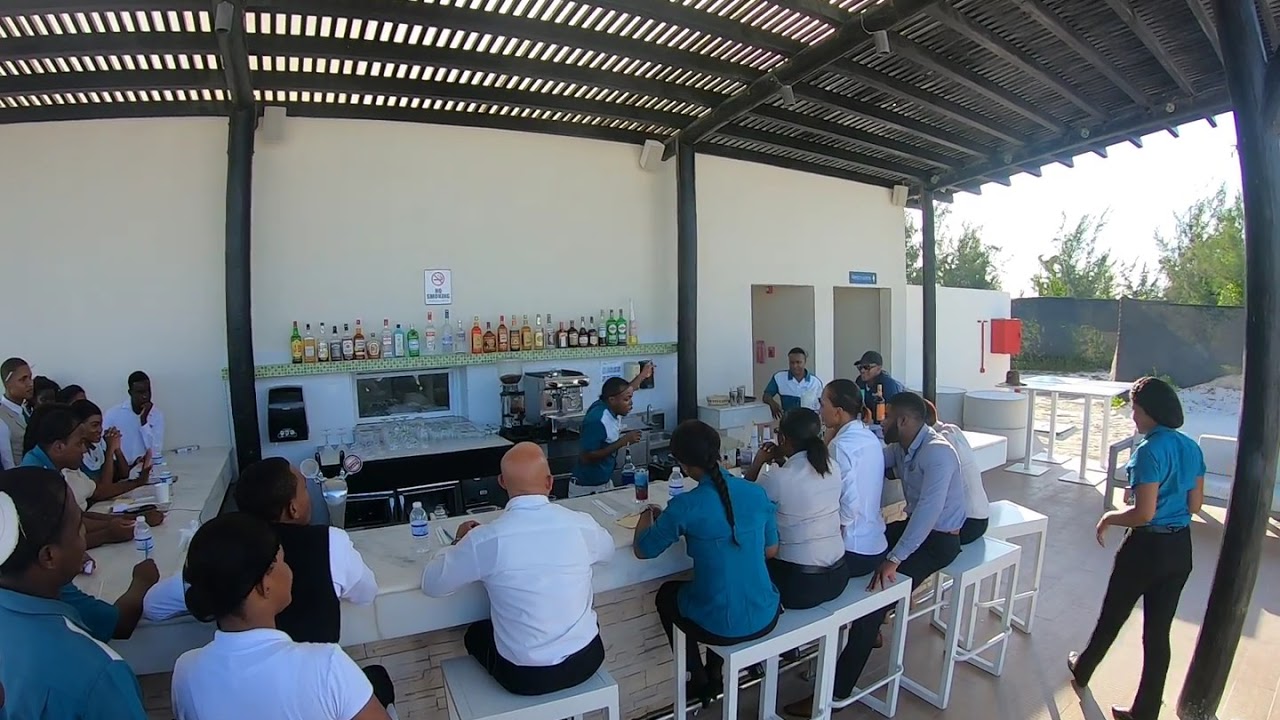The image depicts a bustling outdoor bar and dining area, covered by a metal black awning with wooden slats that provide partial shading. In the mid to late evening light, several people are seated at a long white counter on matching white stools. They have their backs to the camera, with some facing the left where other patrons’ faces are visible. The attendees, a mix of African-American and a few White individuals, are dressed in nicely in white and blue shirts. Drinks such as water bottles and various glasses are placed in front of many of them.

At the back of the counter, a kitchen area with a black stove is visible. A bartender in a blue shirt occupies the open space behind the counter. Behind them, shelves display an array of liquor bottles of different sizes and shapes. Clear glasses are also neatly arranged on another shelf. Further to the right, a waitress, also wearing a blue shirt and black pants, is seen attending the area. A few trees and fencing are present on the right-hand side, indicating that the scene is likely set in the rear of the establishment, enhancing the outdoor ambiance.